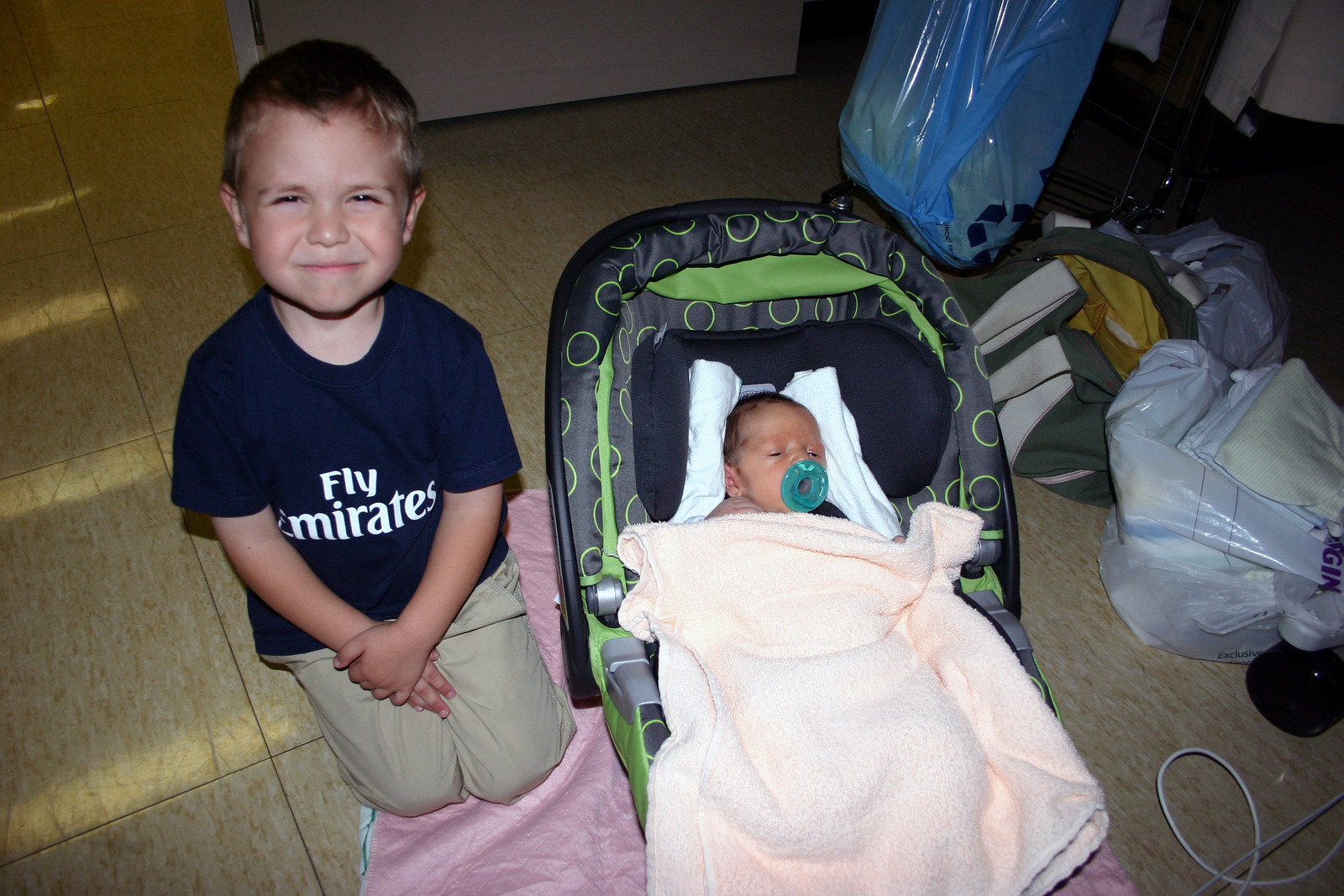In the picture, we see a room with a brownish plywood floor scattered with various items like garbage bags, a blue bag, plastic items, and other unidentifiable objects. In the foreground, a Caucasian little boy with short, brownish-blondish hair, who appears to be frowning or crying, is kneeling on a pink blanket. He is wearing a blue t-shirt that partially reads "Fly Emirates" and khaki pants. His hands rest on his lap as he faces the camera. To the right, a baby with dark black hair is seated in a gray and black car seat adorned with green circles, covered by a peach blanket, and sucking on a pacifier. Sunlight streams into the room, adding to the scene's detail and atmosphere.